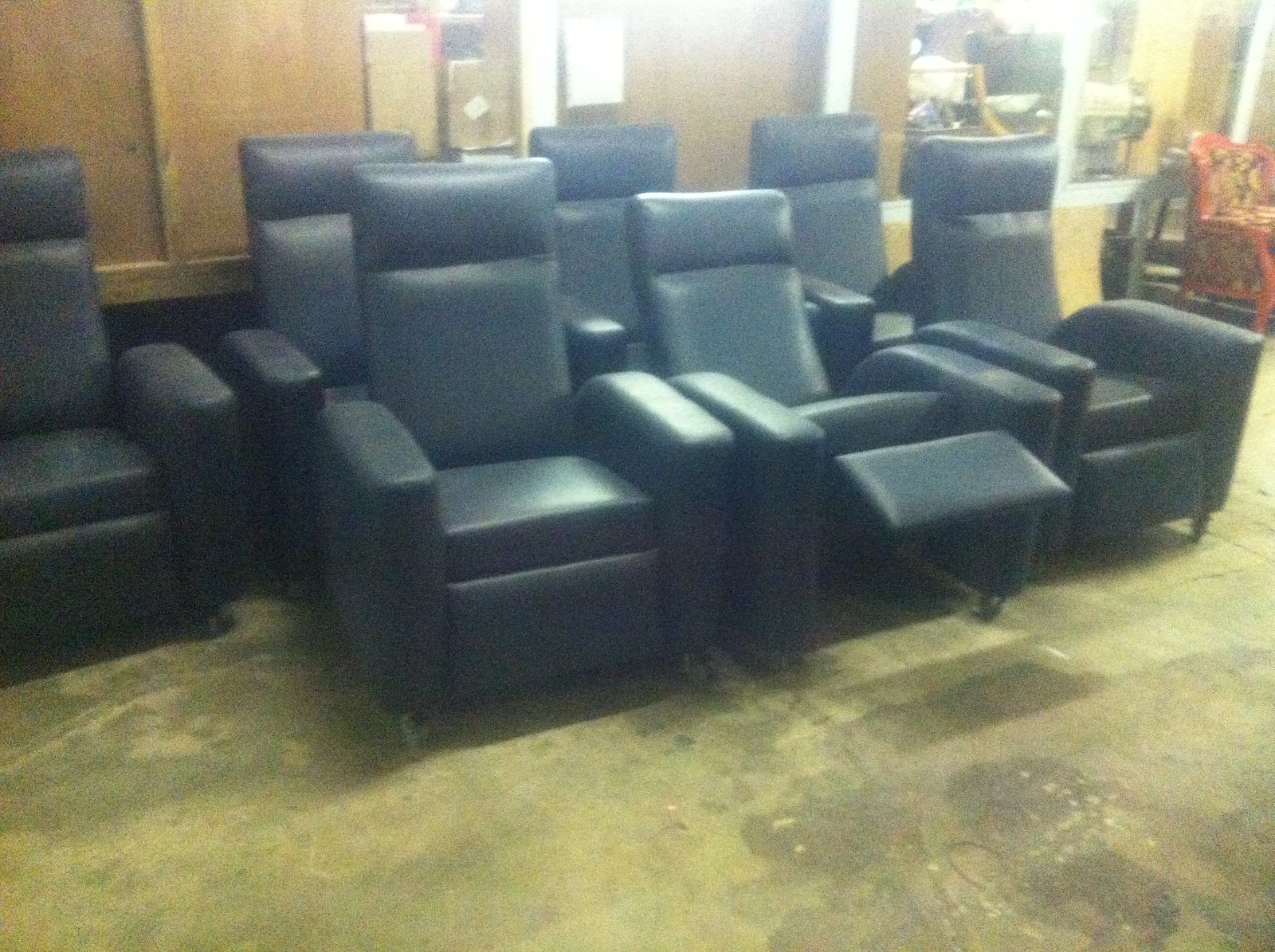The photograph depicts seven identical black reclining chairs, possibly made of leather or a vinyl-like material, arranged closely together in a warehouse or storage room setting. These chairs are polished and have a shiny appearance, with a blackish-blue coloration. One chair in the center of the arrangement has its leg rest extended and its back reclined, while the others remain upright with their leg rests closed. The chairs are positioned on a bare, dirty concrete floor, and the image quality is somewhat fuzzy. In the background, there are wooden walls, bright light entering from an unspecified source, and various pieces of furniture including folding chairs, storage cabinets, boxes, and an easy chair with orange upholstery.